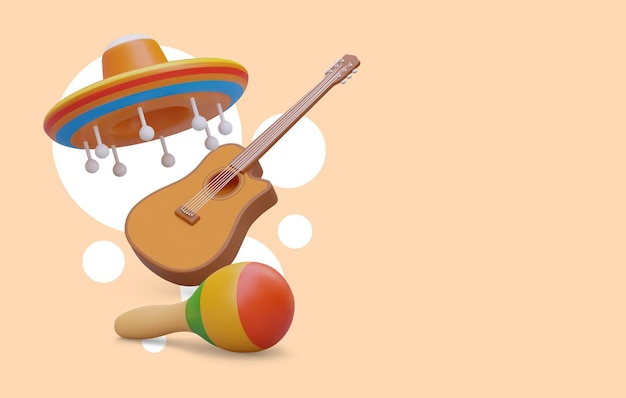This image showcases a digitally created mariachi-themed scene set against a beige, rectangular, horizontal background. At the top of the composition, there is a traditionally styled tan sombrero adorned with blue and red stripes and white tassels hanging from its brim. Positioned directly below the sombrero is a wooden guitar. Beneath the guitar, a pair of wooden maracas are depicted, each featuring a sequence of colorful stripes—green at the bottom near the handle, followed by yellow, and topped with orange. The overall design features abstract white circular shapes, suggesting a simplified, almost cartoonish representation of a mariachi figure. The hat appears to balance precariously over an implied head circle, while the guitar and maracas are positioned as if held by the figure, although they float independently without direct contact. The color palette includes shades of tan, peach, white, light brown, brown, red, green, light blue, and orange, contributing to the festive, vibrant atmosphere of the image.